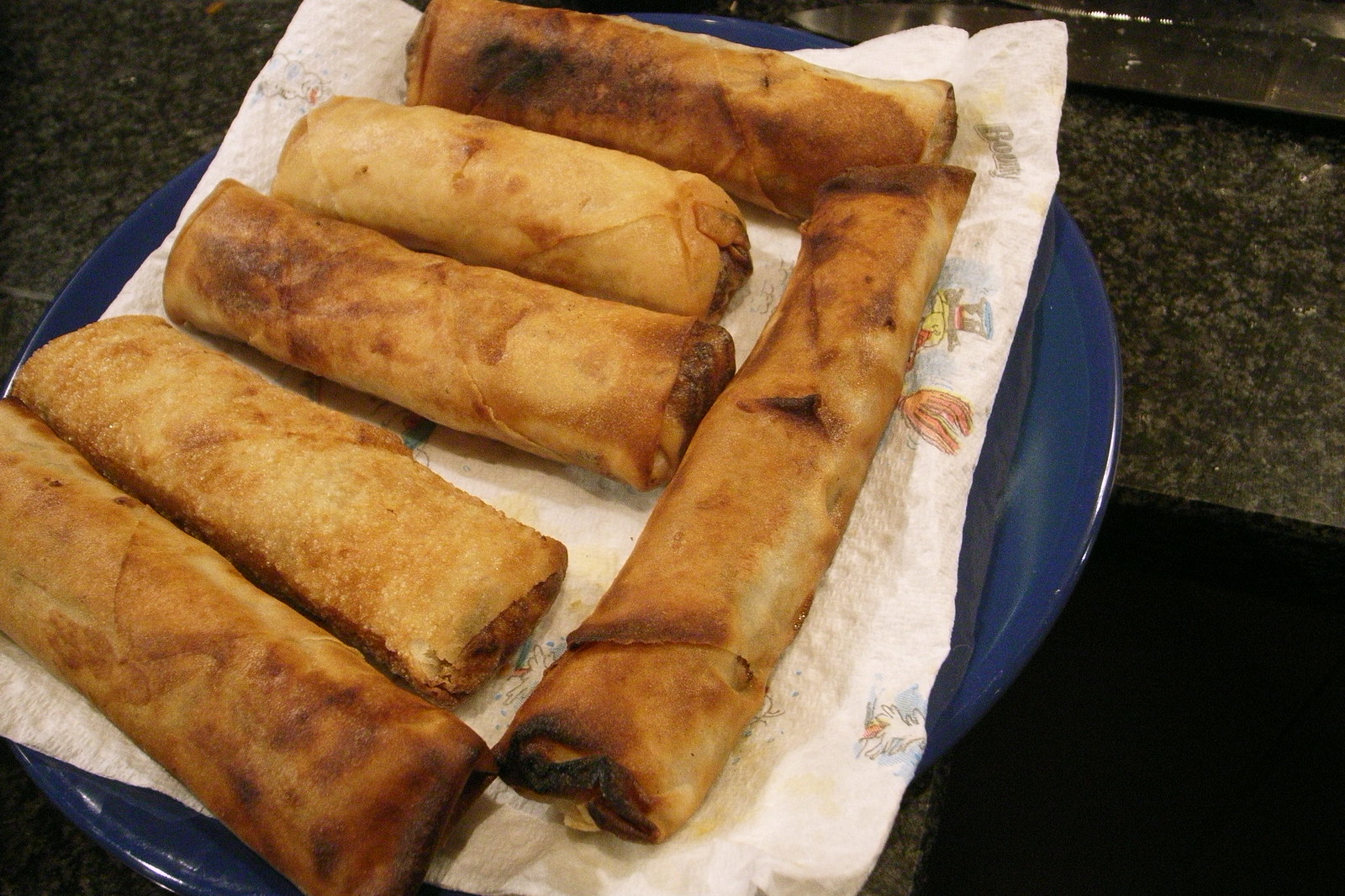The image depicts six cylindrical, fried food items that resemble egg rolls, neatly arranged on a blue, slightly oval plate. These items are nestled on a white paper towel adorned with small cartoon figures and bearing the brand name "Bounty" in the upper right corner. Among the six rolls, one is significantly longer and appears to have burn patches on both ends. Two of the shorter rolls show burns primarily on their ends. The rest are medium brown with darker, almost black areas indicating a crisp, fried texture. The plate is placed on a kitchen countertop characterized by brown hues and granite-like patterns, adding a contrasting backdrop to the food display.